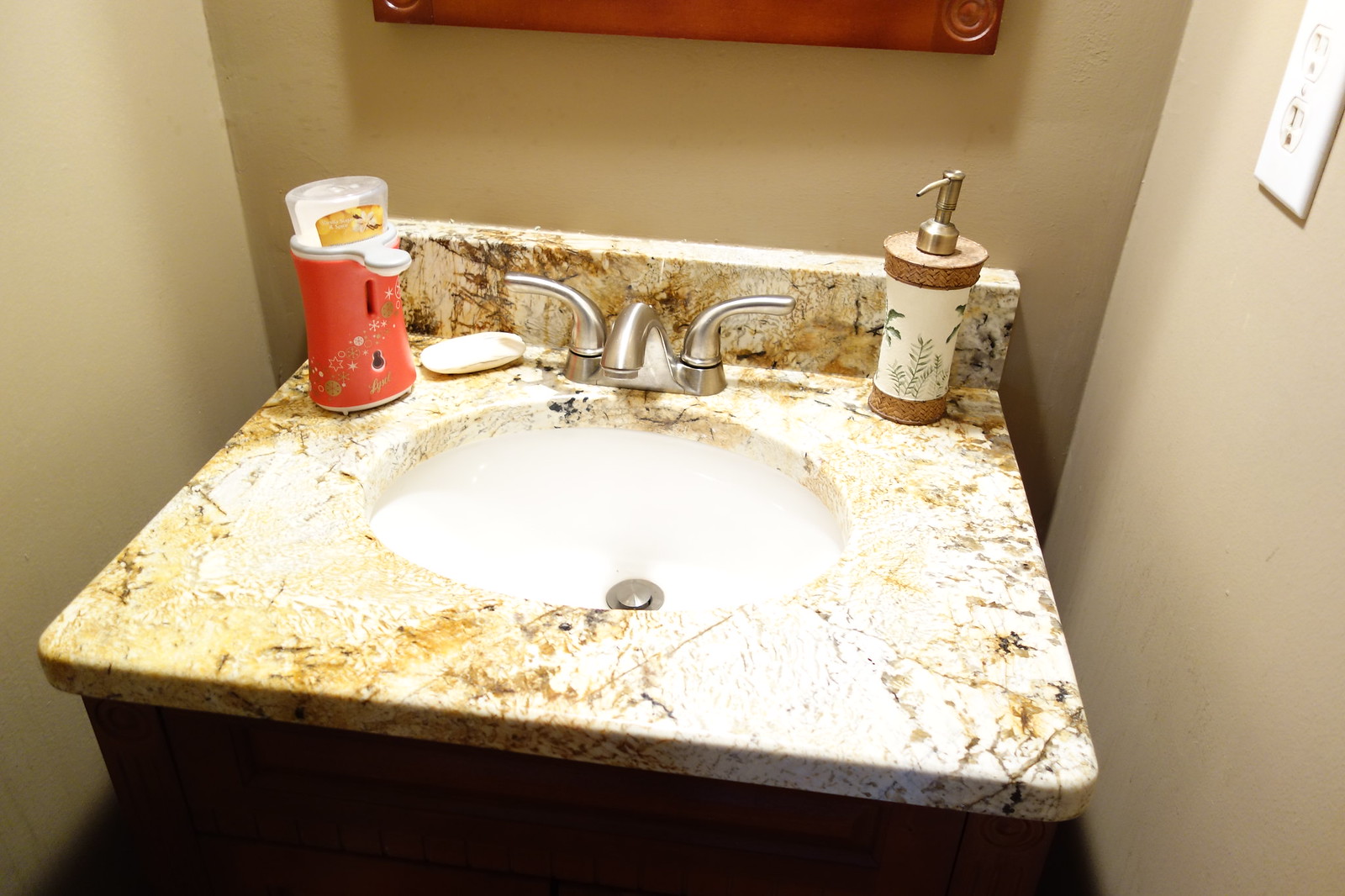This is a detailed color photograph capturing a marble bathroom sink with a white and brown pattern. Although the marble pattern gives the illusion of grime, a closer inspection reveals it's merely the natural design of the stone. The bathroom walls are painted in a light brown hue, complementing the earthy tones of the space. At the top, near the center, part of a mirror frame made from brown wood is visible, hinting at a larger reflective surface just out of the frame. The sink features sleek silver-colored faucets and handles, with the basin's stopper left in the open position.

To the left of the faucets sits a distinct red square object with a clear cap, featuring a circular protrusion. The red container is adorned with diagonal stars in white and gold, and bears the brand name "Lysol" at the bottom in gold script. Beside this, a white bar of soap rests directly on the marble sink top.

On the right side of the faucet stands an elegant hand soap dispenser. This dispenser boasts a stylish brown rattan pattern on its top and bottom sections, while the central part displays a white leafy design. The dispenser's pump is an attractive gold color, adding a touch of sophistication to the overall setup.